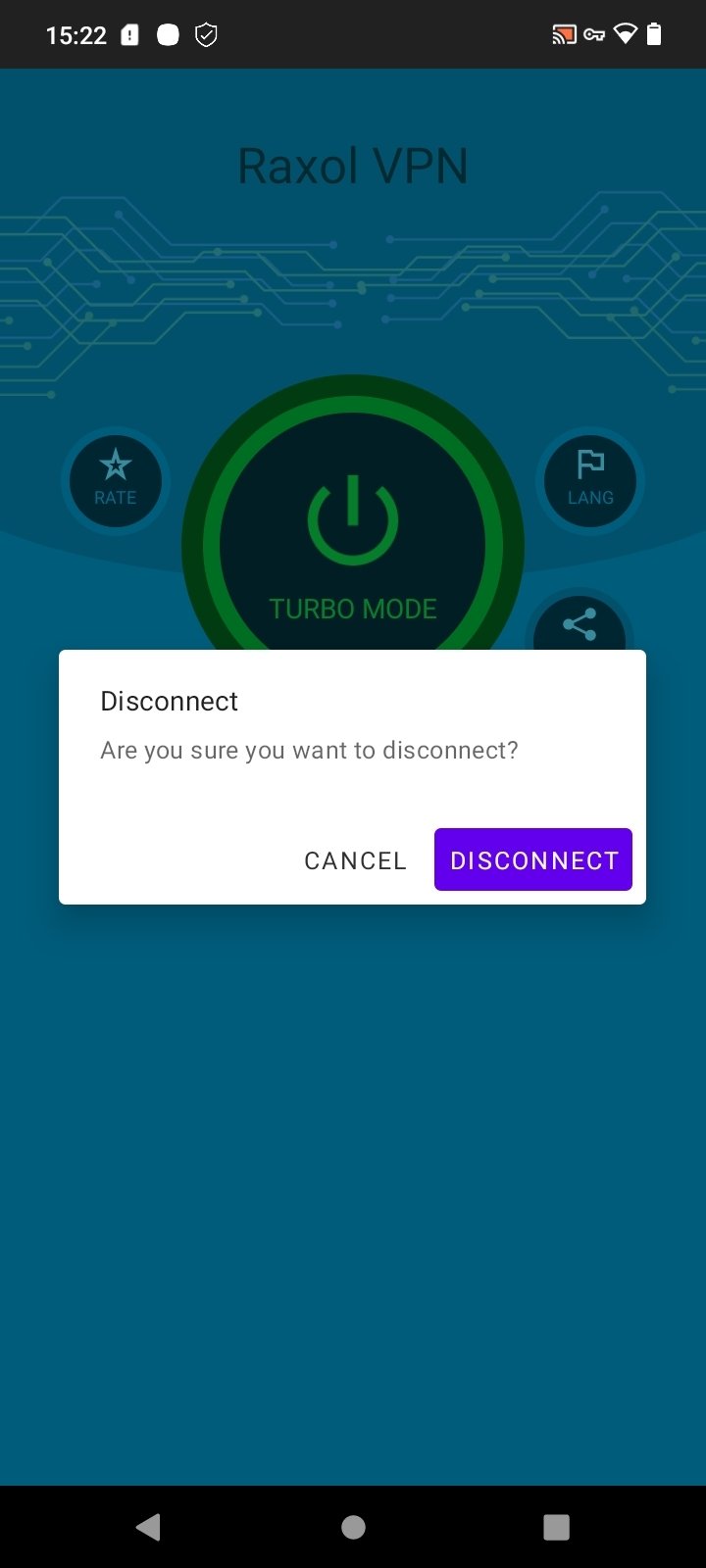This digital screenshot features the Raxel VPN interface at 15:22 military time. The background is blue, providing a calming backdrop to the various interface elements. At the top of the screen, icons indicating a lock, battery status, and Wi-Fi connectivity are displayed. 

Central to the interface is the "Turbo Mode" button, colored green and black with a prominent power symbol, suggesting an enhanced performance mode. Adjacent to it, you can find a "Rate" button symbolized by a star, and a "Language" button marked with a flag indicating the option to change the interface language.

The focal point of the screenshot is a popup window asking the user to confirm disconnection with the message, "Disconnect. Are you sure you want to disconnect?" Below this query are two buttons for the user's response: a "Cancel" option and a "Disconnect" button, distinguished by their purple and white color scheme.

At the bottom of the screen are standard navigation keys: a left arrow button for going back, a circular "Home" button situated in the middle, and a gray square button positioned to the right.